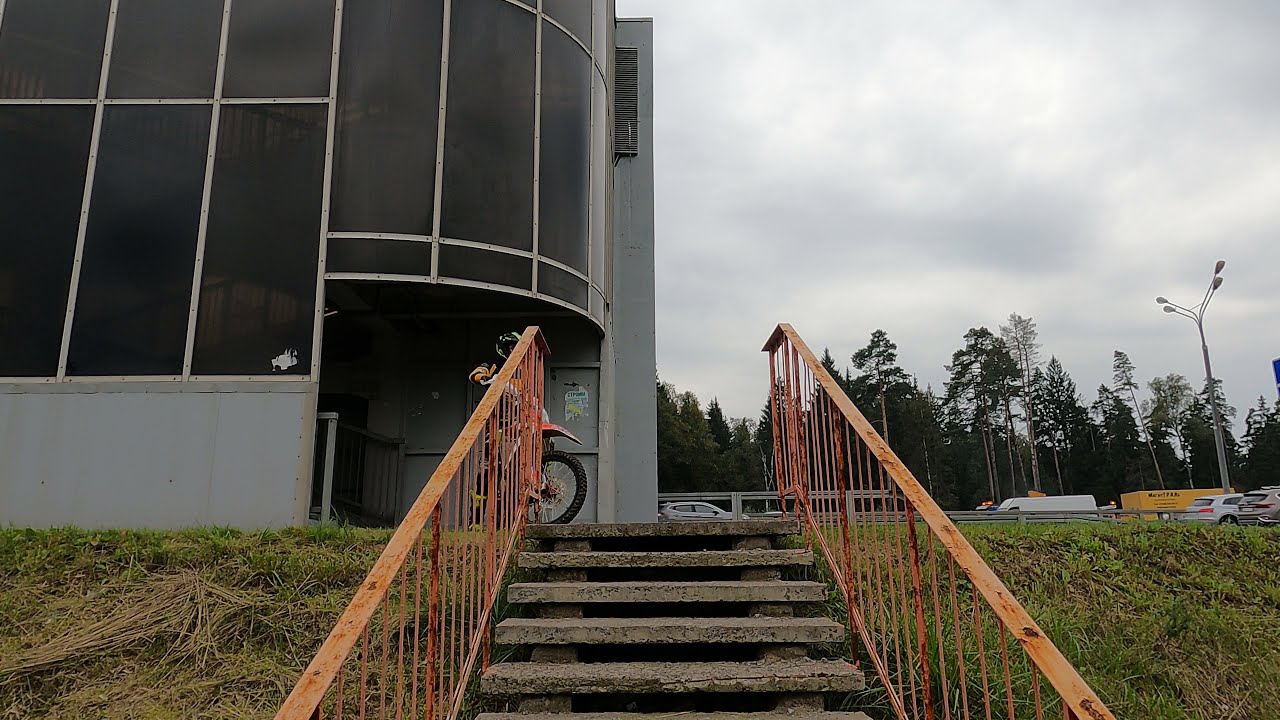This outdoor photograph, taken on a cloudy day, captures a slightly rundown concrete staircase leading to an office-like building on the left. The staircase features orange metal railings, and the surrounding grass is a mix of green and dull brown. At the top of the stairs, there is a non-motorized dirt bike with someone wearing a dark helmet, partially obscured by one of the railings. The building has dark, almost black windows and a gray outer structure, giving it a somewhat dilapidated appearance. In the background to the right, a parking lot filled with cars and trucks is visible, along with a scattering of large green trees and a light post. The sky is overcast, adding to the dreary atmosphere of the image.